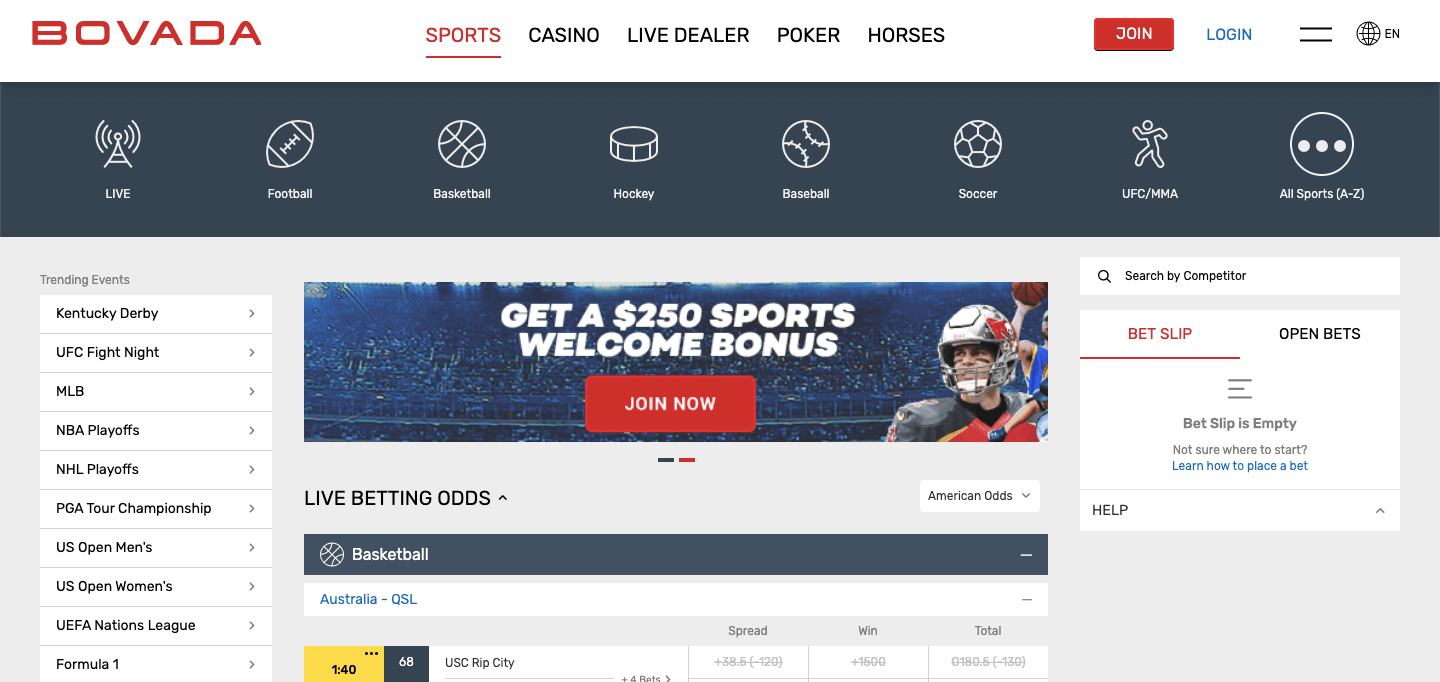The screenshot, likely taken from a laptop in landscape mode, appears to display a section of the Bovada website. The top stripe of the site spans from left to right with a white background. On the top left, the word "BOVADA" is prominently featured in red font. 

Next to the logo, on the same row, are the header options: "Sports," "Casino," "Live Dealer," "Poker," and "Horses." The "Sports" option is highlighted in red and underlined, indicating that it is the currently active page. In the upper right corner, there is a red button labeled "Join," a blue link labeled "Log In," and a globe icon with a dropdown indicating language options, currently set to "English."

Beneath this is a stripe with a black background featuring various icons associated with different live sports: "Live," "Football," "Basketball," "Hockey," "Baseball," "Soccer," "UFC," "MMA," and "All Sports A-Z."

The main content below this banner is divided into three columns. The left column lists "Trending Events" with expandable rows for events like the Kentucky Derby, UFC Fight, MLB, NBA Playoffs, NHL, PGA Tour, US Open, US Open Women's, UEFA Nations League, and Formula One.

The center column starts with a large, vibrant image of an arena, highlighting a promotional offer for a "$250 Sports Welcome Bonus." This image includes various athletes from different sports, featuring a prominent football player. Beneath this image is a large red "Join Now" button. Below this banner, there are rows labeled "Live Betting Odds" and "American Odds," followed by details on a basketball match under "Australia QSL."

The right column contains a search bar with the prompt "Search by Computer," and below it, a section labeled "Bet Slip," highlighted in red. Currently, the bet slip is empty, accompanied by a note encouraging users to learn how to place a bet.

This detailed layout and categorization help users easily navigate through various sports events and promotional offers on the Bovada website.